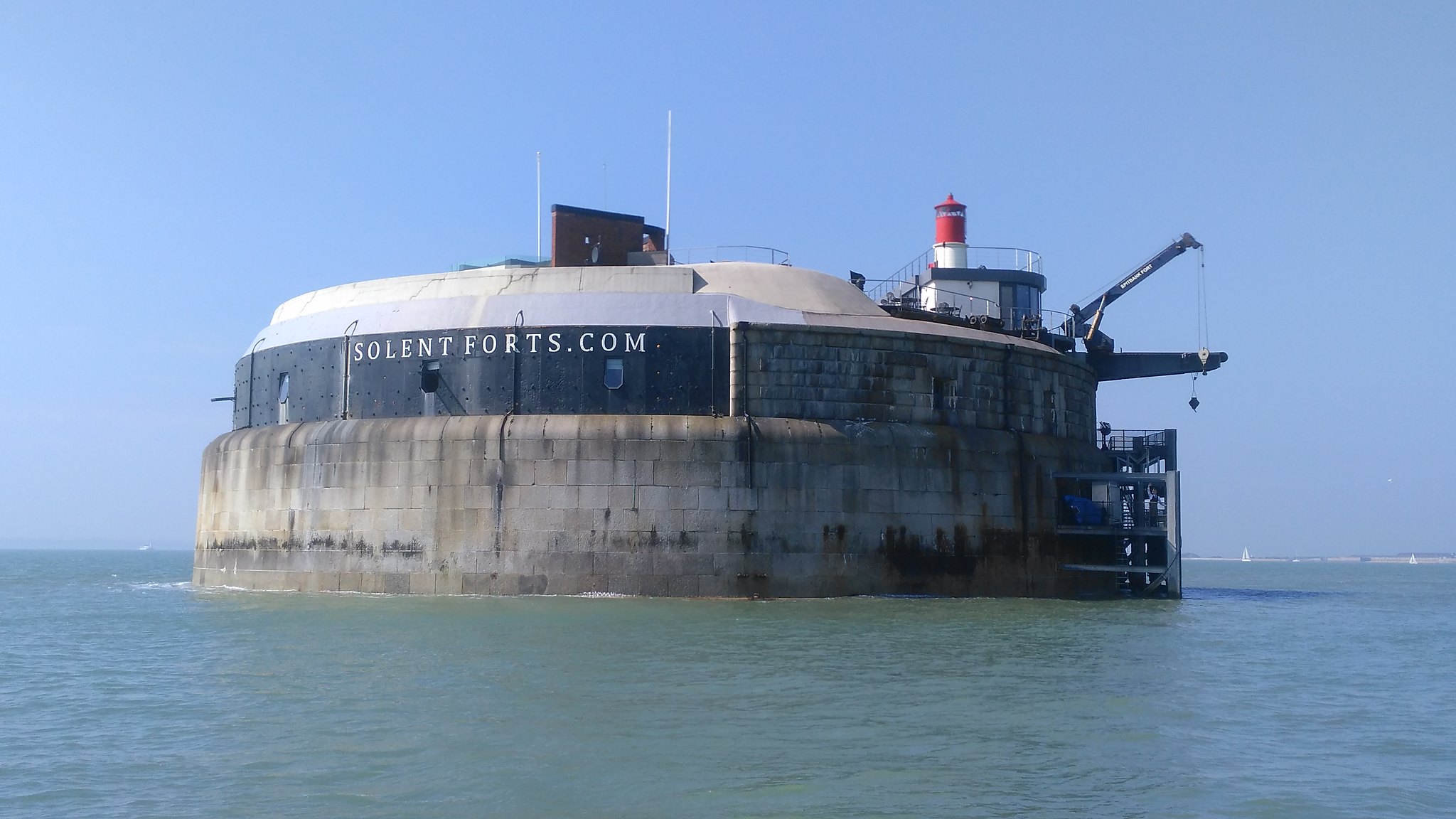This image captures a historic fort in the Solent, near Portsmouth, likely taken from a boat positioned on the surrounding waters, either a large lake or the ocean. This fort, advertised as Sollentforts.com, appears to have been repurposed into a site of interest, potentially a luxury hotel or museum. The structure, built into the water on a concrete foundation, rises several tens of feet above the surface, resembling an artificial island. It exhibits a navy blue lower section and a white upper section, complete with a circular turret and a red-and-white lighthouse perched on top. Protruding from one side is a crane, along with a stairway allowing access from the water. Additional features include flagpoles, antennas, and a vertical wall, enhancing the industrial yet historic aesthetic of the fort.